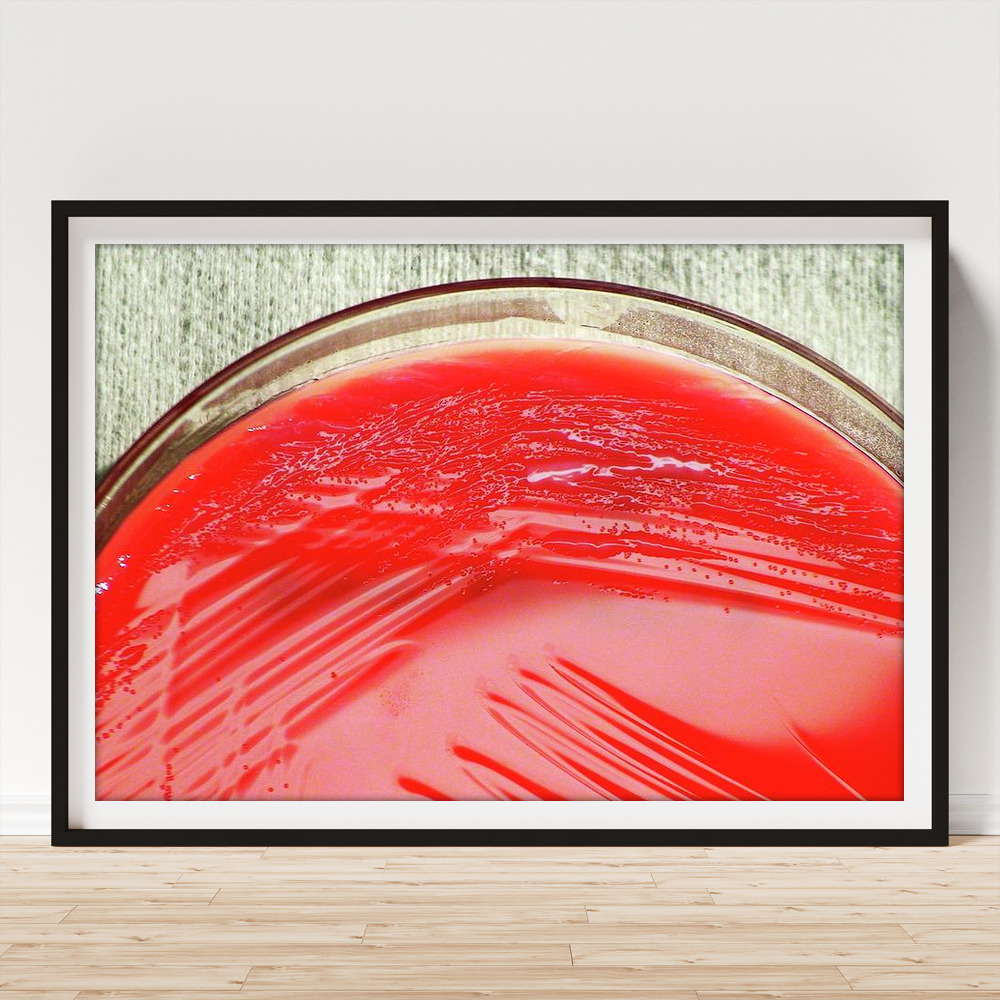The image is a photograph of a striking piece of art with a black frame and a white mat, leaning against a white wall. The floor beneath is a light-colored wooden surface. The artwork captures a top-down view of a glass bowl filled with a red, gelatinous substance, likely resembling red jello, with reflections and ripples suggestive of plastic wrap covering it. The bowl's oval contour stretches from the middle left to the top right, accentuating the vibrant red contents within. The background features a gray, cloth-like texture with vertical striations, encased within a gray border that adds depth to the presentation. The entire composition is meticulously framed, making the red hues in the glass bowl stand out brilliantly against the monochromatic tones surrounding it.